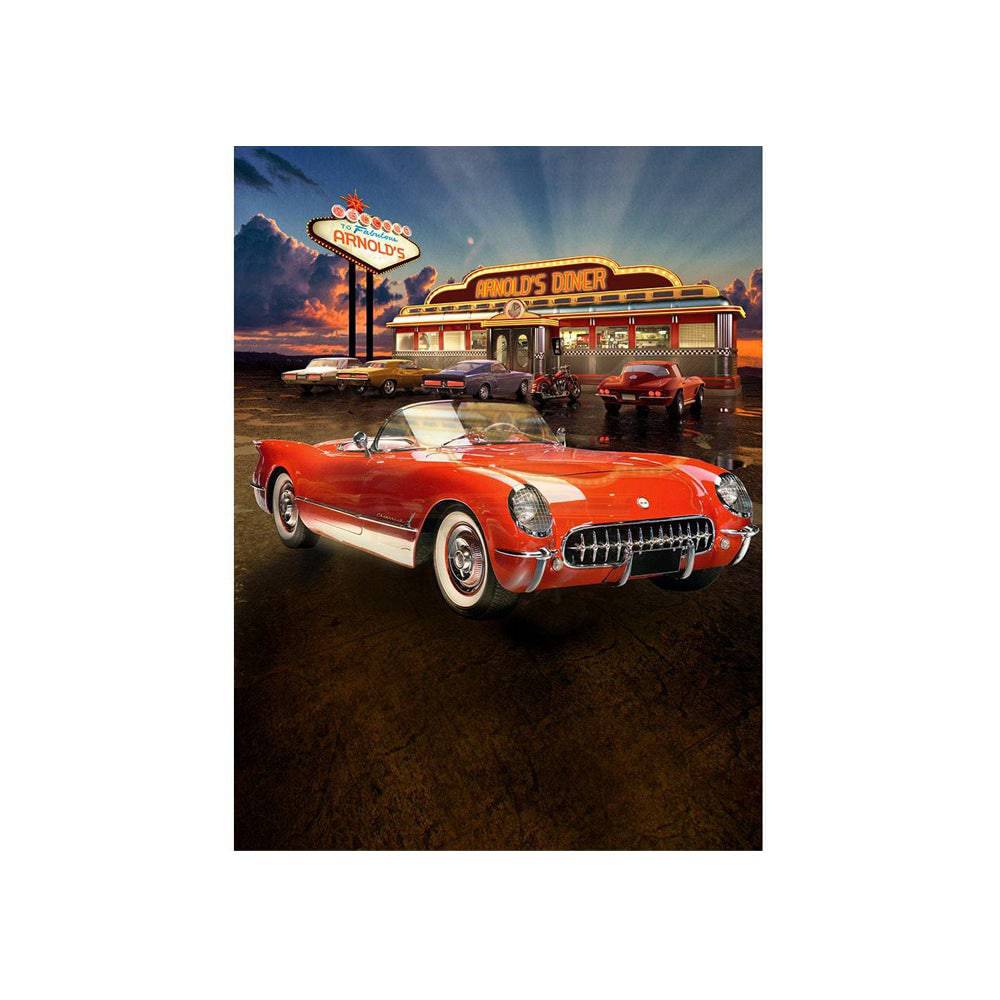The photograph depicts a lively scene at Arnold's Diner, where the setting sun casts a dark blue evening sky with dramatic beams of light peeking through the clouds. The centerpiece of the image is a pristine red convertible sports car, positioned prominently in the foreground with its sleek, shiny body and top-down configuration, reflecting the waning sunlight. The diner itself appears nostalgic, built from a vintage streetcar or train, featuring stainless steel sides and classic streetcar windows. Above its double door entrance, a sign reads "Arnold's Diner," while to the left, another sign fashioned after the iconic Las Vegas sign proudly displays "Welcome to Fabulous Arnold's." Adding to the retro ambiance, the diner’s parking lot showcases four polished old-fashioned cars facing the diner and a red motorcycle, all lined up on the brown cement pavement.